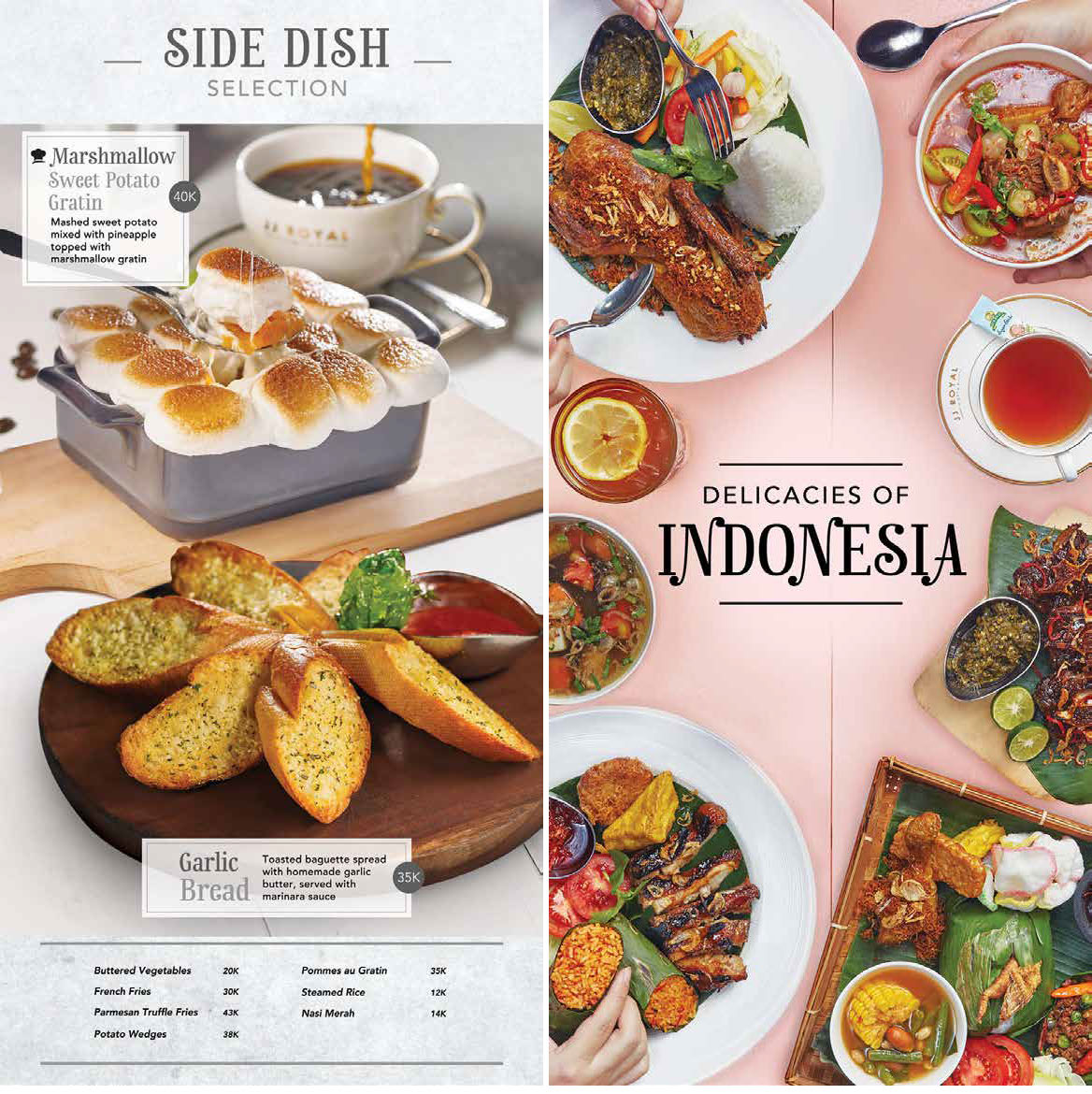The flyer is a promotional material for a restaurant, divided into two distinct sections. On the right side, titled "Delicacies of Indonesia," there are various dishes depicted, arranged around the central text. The dishes feature an assortment of foods such as different types of meat, rice, vegetables, and sauces, each presented in individual plates. Additionally, there are two cups of tea: one hot and one iced, the latter garnished with a lemon slice. Above this section, a fork and spoon positioned next to a hat suggest readiness to dine.

On the left side of the flyer, the section labeled "Side Dish Selection" showcases more food items with detailed descriptions and prices. The topmost image is of a cup of coffee being poured into a saucer with a spoon beside it. Below that, a wooden platter holds garlic bread, labeled clearly under the plate. The description notes that it is a toasted baguette spread with homemade garlic butter, served with marinara sauce for 35k. Another dish shown is marshmallow sweet potato gratin, which includes mashed sweet potato mixed with pineapple and topped with a marshmallow gratin, priced at 40k. Additional side dishes listed include buttered vegetables for 20k, french fries for 30k, parmesan truffles for 43k, potato wedges for 38k, pommes al gratin for 35k, steamed rice for 12k, and nasi merah for 14k.

This carefully arranged flyer not only visually highlights the appeal of the restaurant's offerings but also provides detailed descriptions to entice potential diners.